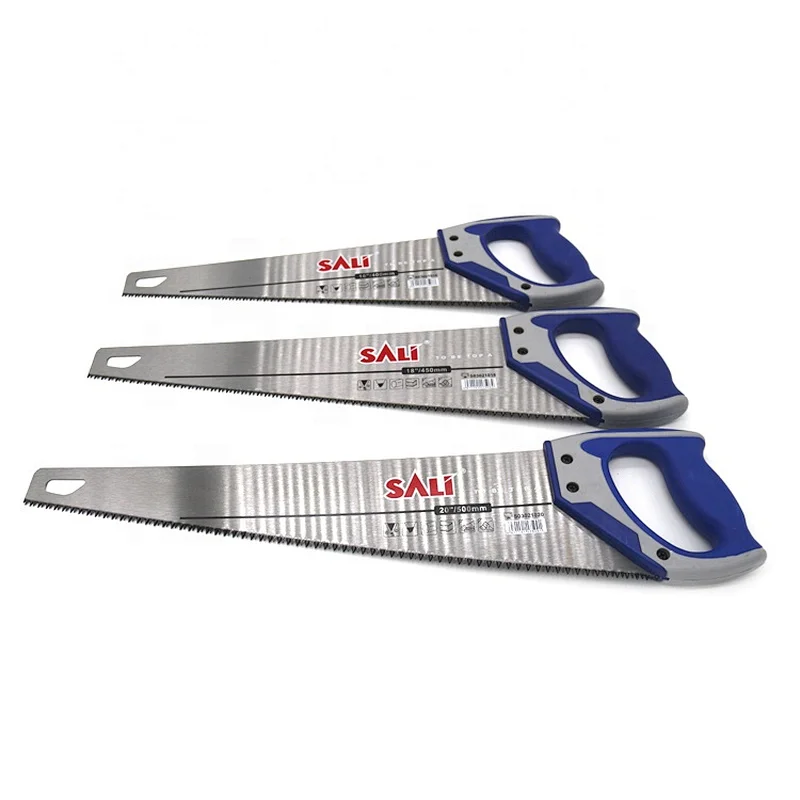Displayed against a plain white background, the image shows three hand saws arranged vertically in a row, with the largest saw at the bottom and the smallest at the top. Each saw shares the same model design but varies in size. The handles, positioned on the right side of the saws, feature a combination of blue grips and gray connections to the blades, each secured with three black screw holes. The saw blades are shiny silver metal with a consistent design across them.

The branding "SALI" is prominently written in red letters with a white outline on the upper half of each blade. Below the brand name, a black horizontal line stretches from the handle to the tip of the blade. Further below, various texts describe the saw size, the barcode is found on the right side, and illustrations on the left side depict the materials the saws are capable of cutting. A distinctive hole is located near the tip of each blade, emphasizing the consistent design features among the differently sized saws.